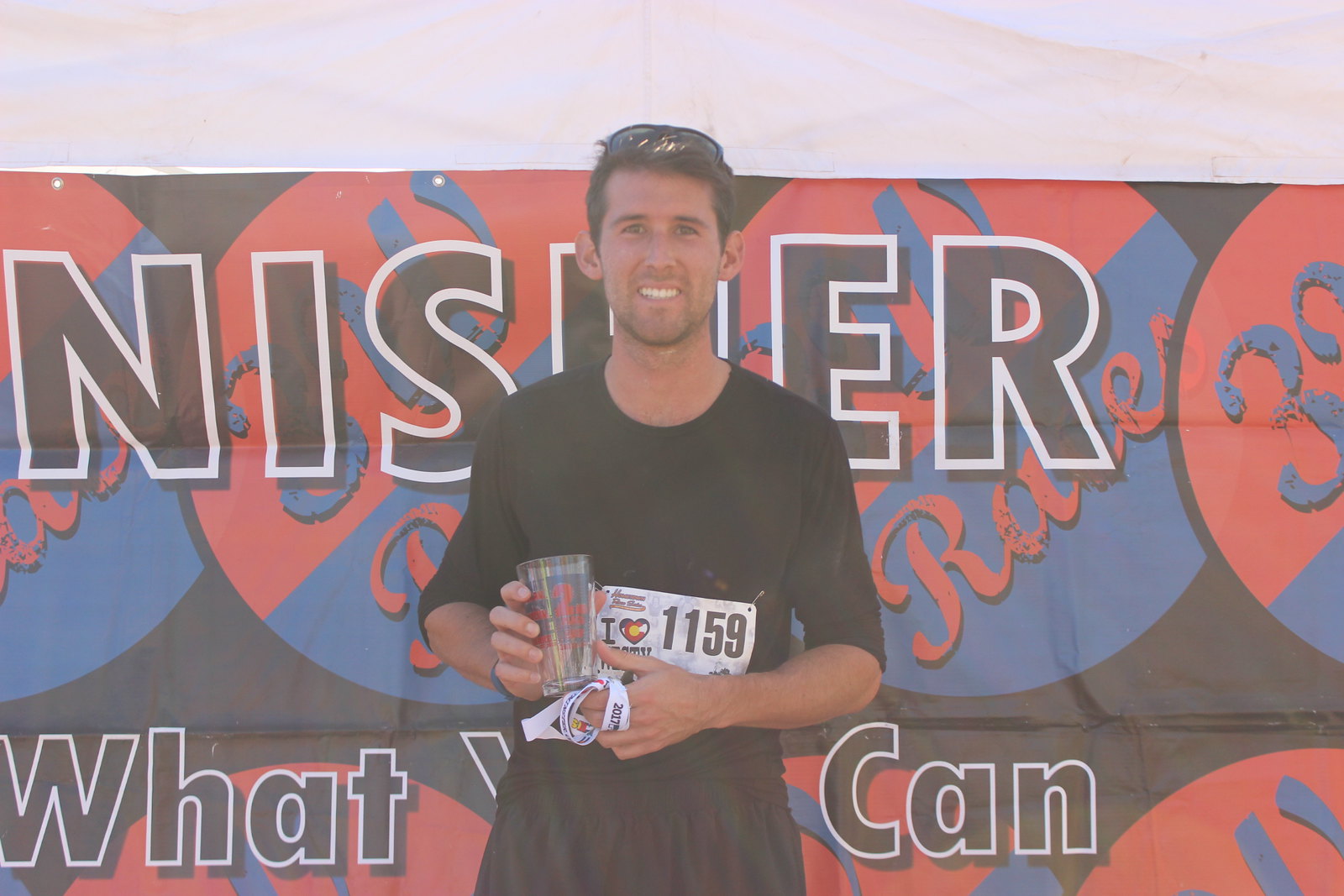In this photograph, set in landscape mode and slightly over-processed with a faint tan filter, a man in his mid-20s stands front and center, exuding a proud and happy demeanor. His white skin has a tanned hue, and his short brown hair is adorned with black sunglasses perched on top. His ears slightly protrude, and he sports a half-smile, revealing the top row of his teeth. He wears a black, short-sleeve t-shirt with a crew neck and black shorts or pants. His right hand holds a plastic cup emblazoned with a bold red "2" and unreadable text, while his left hand has a lanyard wrapped around it, displaying the year "2017." A white sign with the numbers "1159" is draped across his stomach, partially obscuring the words "I love" on his shirt beneath. Behind him, a white banner with red and blue circles and partially legible text that reads "KNISER" and "what you can" adds to the backdrop. The image captures a moment filled with cheerful energy amidst a bustling event.